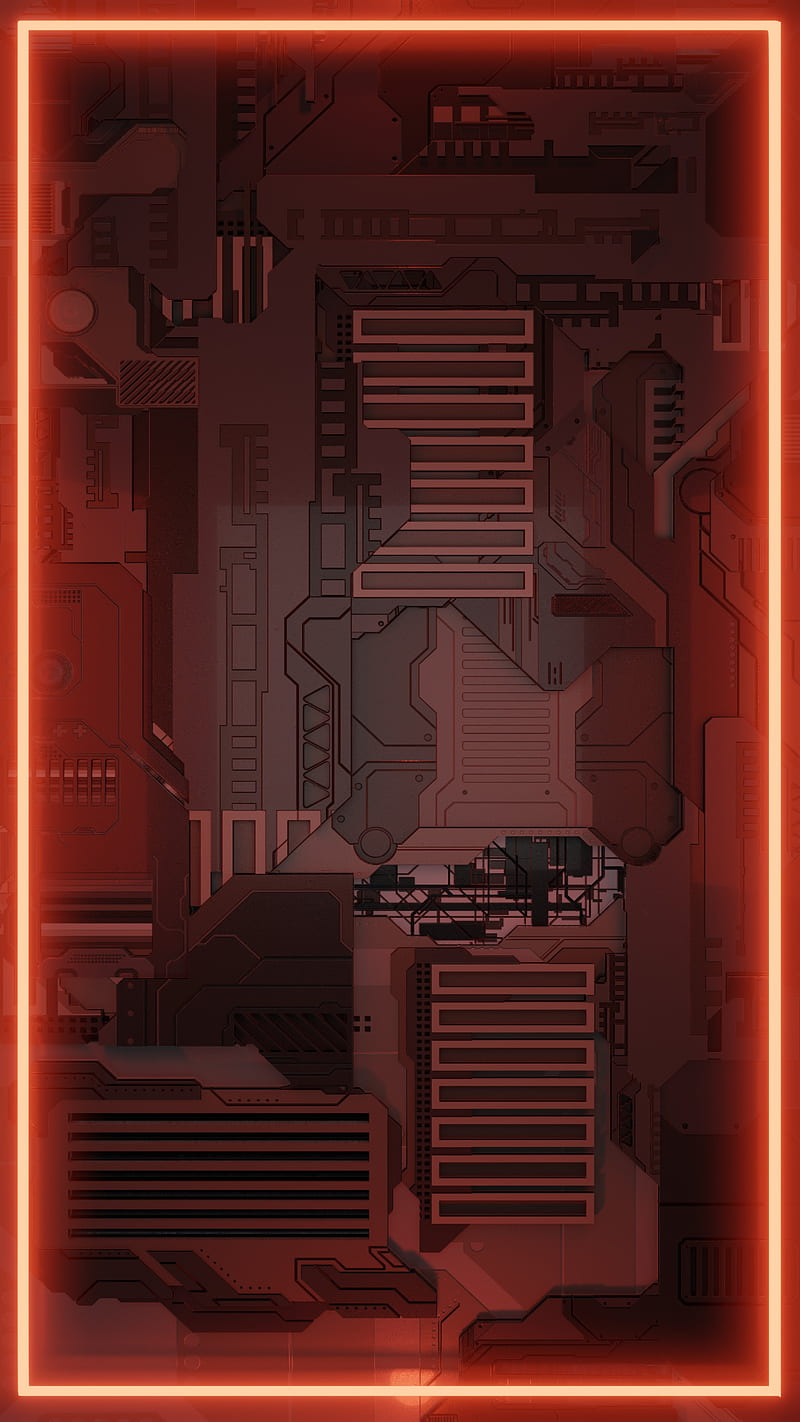The image depicts a highly stylized digital artwork that combines elements of both a sketch and a computer graphic. The scene appears to be the interior of a futuristic room, predominantly rendered in black, gray, and darker gray tones, accentuated by a vibrant, glowing red border that frames the entire composition. This red border emits a neon-like glow, creating a striking contrast against the darker elements within. Inside the frame, various geometric, rectangular shapes—resembling modern shelves or drawers—are arranged in a vertical stack, evoking the appearance of a wall adorned with high-tech knickknacks or tools. These shapes exhibit a reddish hue with black interiors, adding to the modern, high-tech aesthetic. Additionally, intricate, high-tech wiring can be seen, contributing to the overall impression of a circuit board or a digitized room. The background also features a window-like element and a notable detail: the number '100' is subtly inscribed in the bottom left corner. Overall, the digital image combines futuristic design with elements that evoke the structured complexity of a circuit board, encapsulated within a glowing, red-bordered frame.